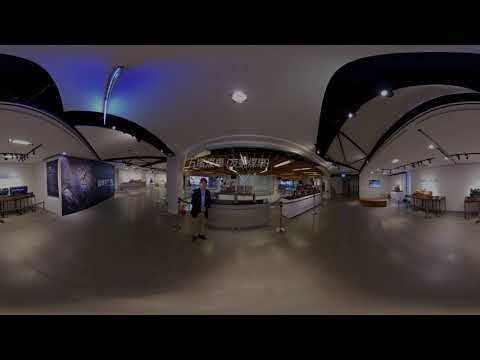The interior image appears to be taken with a fisheye lens, giving it a rounded, slightly distorted perspective. The setting seems to be a public, commercial space such as a mall or theater. Dominating the center of the image is a gentleman wearing khaki pants, a dark blue blazer, and a light blue shirt, standing in front of what looks like a counter or desk area. The counter could potentially be a bar or a ticketing area, and is flanked by chairs against whitish, curved walls. There are horizontal lines framing the darker ceiling at the top and bottom of the image. To the left, there's a blue light casting a glow, possibly illuminating an art display or large signage panel. On the right, white lighting highlights tables against the wall. Additionally, there appears to be stanchions or separation poles in the center-right of the image, reminiscent of crowd control barriers in a movie theater.